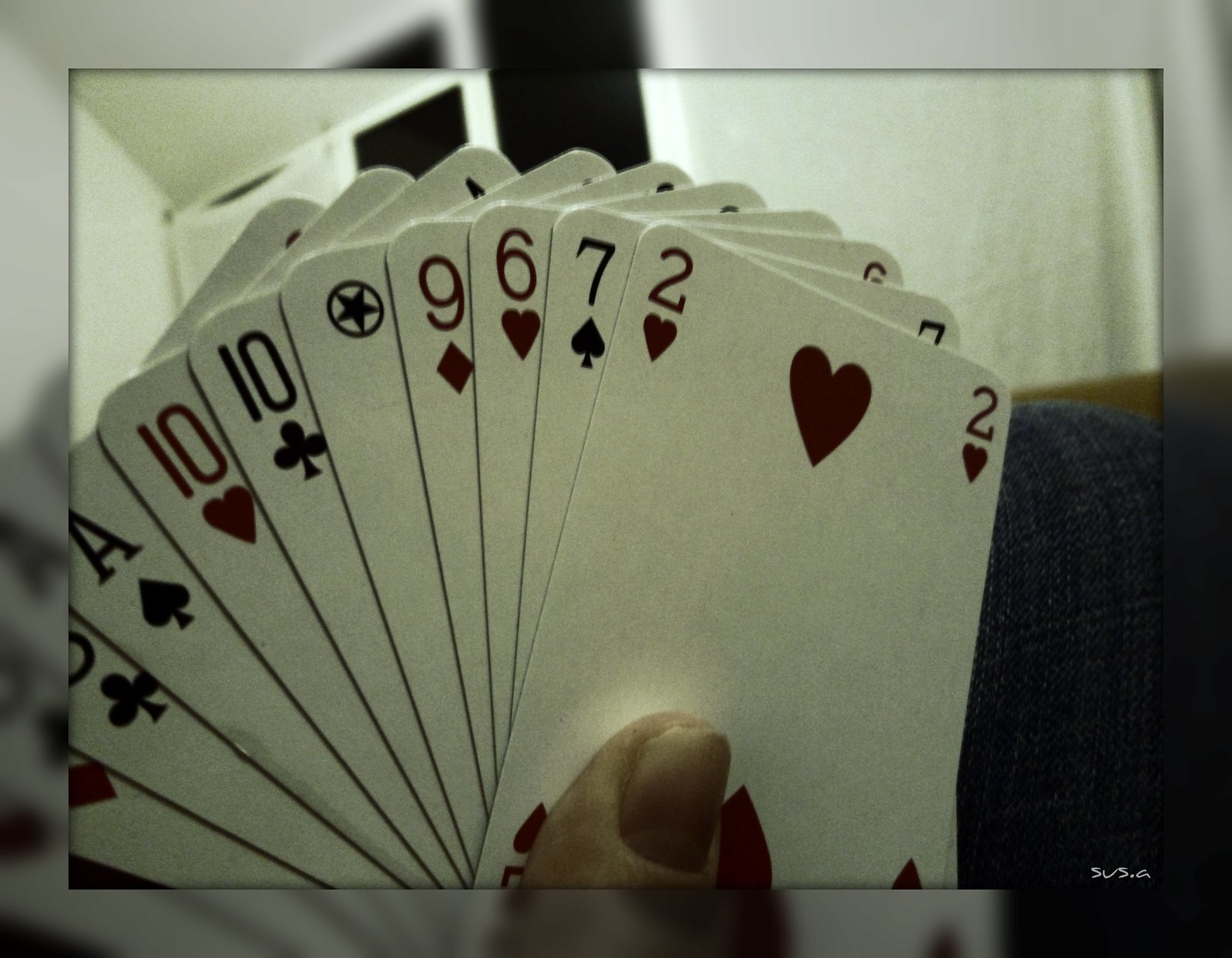This photograph captures an image of a hand holding a fanned-out set of playing cards against a backdrop of what appears to be a denim fabric. The visible cards include the 2 of Hearts, the 7 of Spades, the 6 of Hearts, the 9 of Diamonds, and the 10 of Clubs, alongside a couple more with a 10 of Hearts and 8 of Spades partially visible. There is also a unique card featuring a simple black star icon. The person's thumbnail and fingernails, painted in a light pink shade with darker pink details, are clearly visible as they hold the cards. 

The image has a watermark at the bottom with white font, which seems to spell out "SUSG." In the background, you can see a white wall and part of a door, reflecting some overhead lighting. There is a square frame effect around the photograph which gives off a hint of color from the photo behind it.